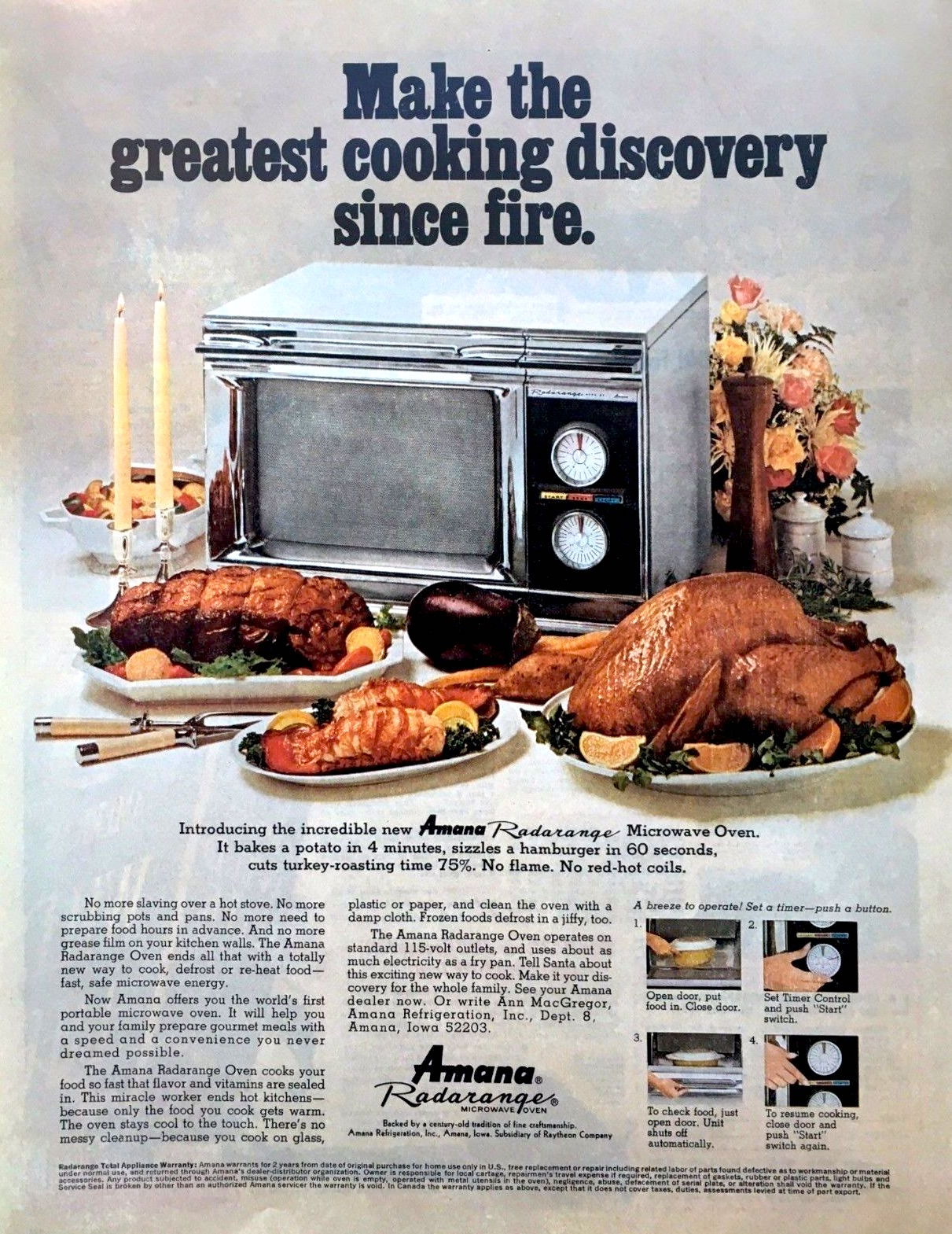This vintage magazine advertisement features a color printed, vertically oriented image showcasing the groundbreaking Amana Radar Range microwave oven. At the top, bold black text proudly proclaims, "Make the greatest cooking discovery since fire." Below this headline, the star of the ad, a sleek, chrome-finished microwave oven with two rounded white dials on the right side, takes center stage. Arranged around the microwave are a variety of freshly cooked foods, including a turkey on a platter garnished with orange wedges, and multiple other dishes that highlight the microwave’s cooking capabilities. 

In the background, decorative elements such as flowers, salt and pepper shakers, and two lit candles add a homely touch. The advertisement's subhead introduces the "incredible new Amana Radar Range microwave oven," boasting impressive features like baking a potato in four minutes, sizzling a hamburger in 60 seconds, and cutting turkey roasting time by 75%, all without the need for flames or red hot coils.

The lower part of the page includes additional details, with smaller text detailing more features and benefits of the microwave, although it is too small to read clearly. Four smaller, detailed color photographs of the microwave’s control panels are displayed on the bottom right, emphasizing the innovative design and advanced technology of the product. The overall aesthetic of the ad is representative of a vintage print publication with a gray background and a focus on the modern convenience of the Amana Radar Range microwave oven.